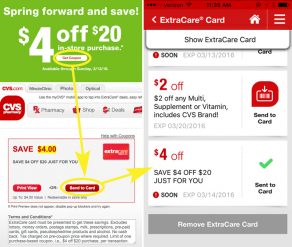The image depicts a mobile screenshot of the CVS Pharmacy app showcasing several digital coupons available to the user. On the left side, there's a prominent green section highlighting a coupon that offers "$4 off $20 in-store purchases." Beneath this, the text "CVS pharmacy shop deals: Save $4" is visible, with a partially legible circled note and an arrow pointing to various other coupons. 

Further down, another coupon reads "$4 off $20 just for you," indicating an additional saving opportunity. At the top of the screen, there's a banner for "$2 off any multi-supplement or vitamin, includes CVS brand," which also suggests that users must show their ExtraCare card to redeem the offer. Options to "Send to card" or potentially remove these offers are displayed, hinting at the functionality within the app to link these savings directly to the user's CVS account for easy redemption. This curated list of discounts reinforces the benefits of using the CVS app for regular customers, providing them with convenient access to numerous savings and promotional deals.